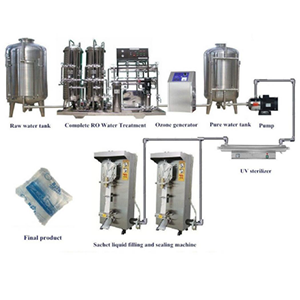The image is a detailed schematic of an industrial process, primarily depicted in gray, blue, and black colors. Central to the illustration is a sequence of large tanks, piping mechanisms, and various pieces of equipment. From left to right, the process appears to begin with a large silver vat, followed by a network of silver pipes leading to another silver and black tank. The next stage involves a silver box with a blue label and a connected canister. A red, white, and black pump is then shown, linking with another apparatus that resembles a vent. Further along, there are two additional pieces of equipment, one on the left and one on the right, interconnected by pumps and additional piping. The rightmost dispenser is a substantial gray box with a white pipe. The process concludes with what looks like a final product encased in a translucent blue and gray container, possibly plastic. At the bottom left of the image, a translucent bag, likely containing ice or a water-softening substance, is visible. Though the detailed blue text under each item is illegible, the overall depiction is of a complex industrial system involving vats, pumps, generators, and a final packaged product.